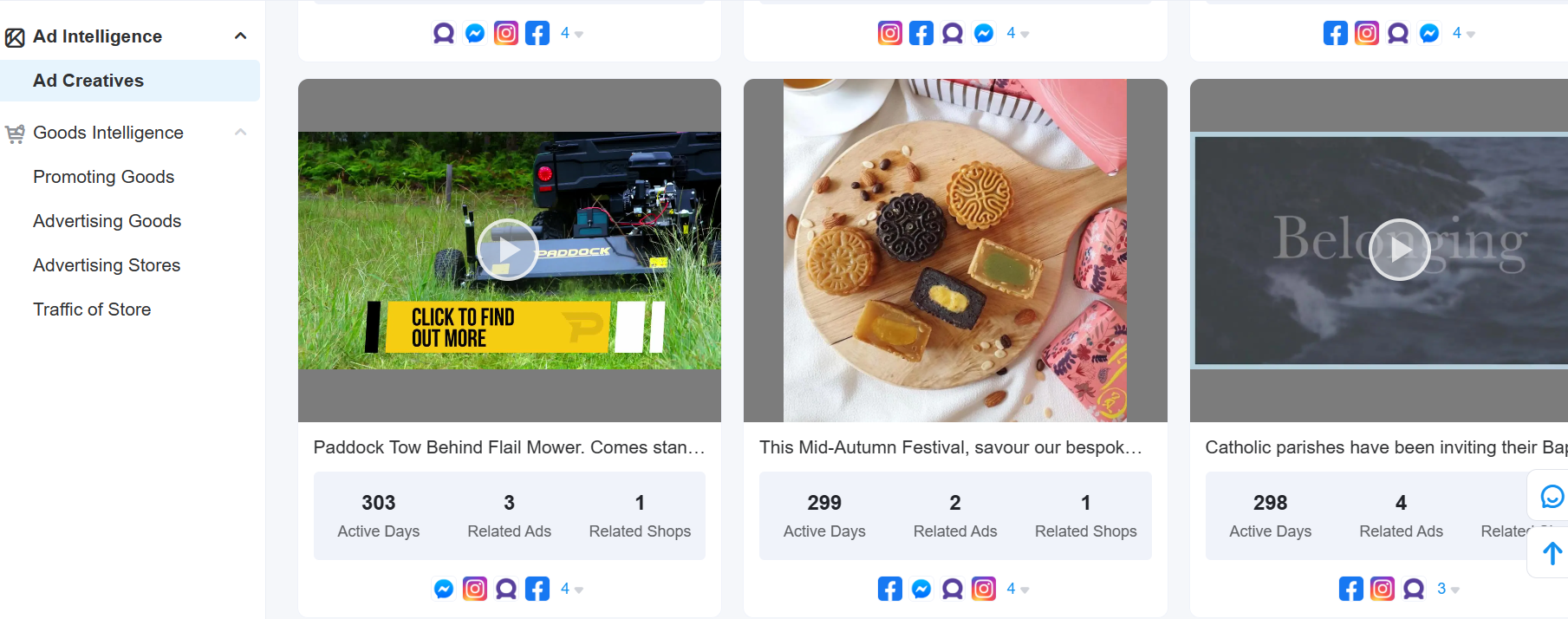In this social media interface screenshot, we see a detailed layout primarily focused on advertising content. On the left side, there's a collapsible column titled "Ad Intelligence" with an upward-pointing arrow, currently highlighted as "Add Creatives."

To the right, three main visual elements are displayed:

1. The first element is a video thumbnail featuring an individual cutting tall grass. A banner across the image reads "Click to find out more," followed by text indicating "Paddock toe behind a flail motor comes stand..." Below this, it mentions "Active days: 303," "Three related ads," and "One related shop." The video thumbnail is marked with a play button in the center, inviting user interaction. The image is bookended by Instagram and Facebook social media icons, depicted as blue squiggly marks above and below the thumbnail.

2. The second element, centrally located, showcases a photo of various cookies and biscuits arranged on a long-handled wooden charcuterie board. A caption below the image states, "This Mid-Autumn Festival, savor our best bespoke picks," followed by "289 or 299 active days," "Two related ads," and "One related shop." Similar to the first element, this image is framed by the same Instagram and Facebook icons on the top and bottom, enhancing the social media context of the post.

3. The final element is another video thumbnail promoting a Catholic parish event, with an enticing play button in the middle and a caption describing the content. It mentions "298 related..." on the left side under "Add Creatives" and a few advertising categories like "Promoting goods" and "Traffic of store." This video element aligns with the overall theme of social media interaction and advertisements.

The entire interface is unified by a white tab on the left side, maintaining coherence across the diverse advertising content and interactive elements displayed in the screenshot.